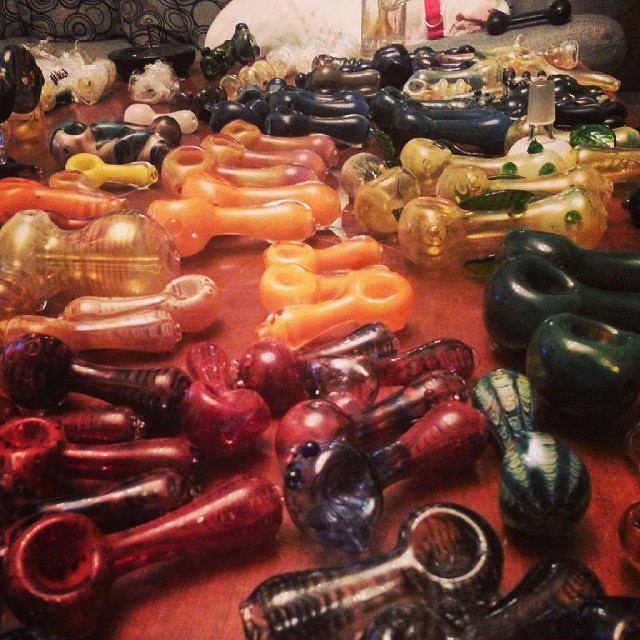The image depicts a reddish-brown table adorned with a collection of uniquely shaped, spoon-like pottery pieces, each featuring distinctive hole-in-the-middle designs. These pieces come in various colors and patterns, including dark green, dark red, and orange hues, as well as gold-lined and gold with green dotted designs. The table holds an array of these thick, plastic-like objects, with some in shades of yellow and black, adding to the vibrant display. In the background, there is a white pillow on a couch, complemented by a gray stone on the right.